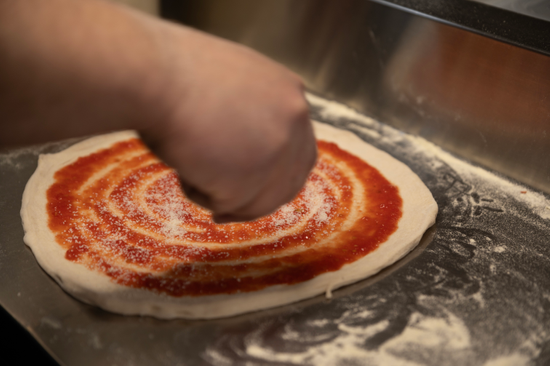In this photograph, a Caucasian individual is in the process of preparing a flatbread, potentially pizza, on a gray prep station. The off-white dough is generously sprinkled with white flour. At the center of the dough, there are circular swirls of red tomato paste, extending outwards and forming gaps that reveal the dough beneath. The person's hand hovers over the central portion, suggesting they are in the act of spreading the flour or adjusting the dough. The outer edges of the dough bear a thicker layer of the tomato paste. The backdrop features a silver metallic surface with a black lip running along the top, adding contrast to the culinary workspace.